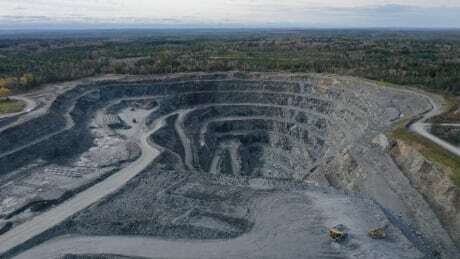This is a rectangular, color photograph taken in landscape orientation, showcasing a large, stepped strip mine set in a remote, undeveloped area. The mine, a circular pit with terraced levels, descends deeply into the ground. The exposed soil of the mine is predominantly grey, with hints of bluish tones. Surrounding the mine, the landscape transitions to vibrant green, indicating vegetation and grass, juxtaposing starkly against the grayness of the mine.

The mine features a complex network of pathways and roadways. A main roadway rings the mine's perimeter, while additional roads spiral downwards, facilitating access to different levels. On the left side of the photograph, a roadway extends from the lower left corner into the mine, following a circular pattern down to the bottom. Towards the front right at the top edge of the pit, large earth-moving machines are visible, highlighting the scale of operations.

Above the mine, a blue sky dotted with white clouds provides a serene backdrop, contrasting with the industrial nature of the scene below. The photograph captures both the grandeur and the meticulous construction of the mine within its natural surroundings.